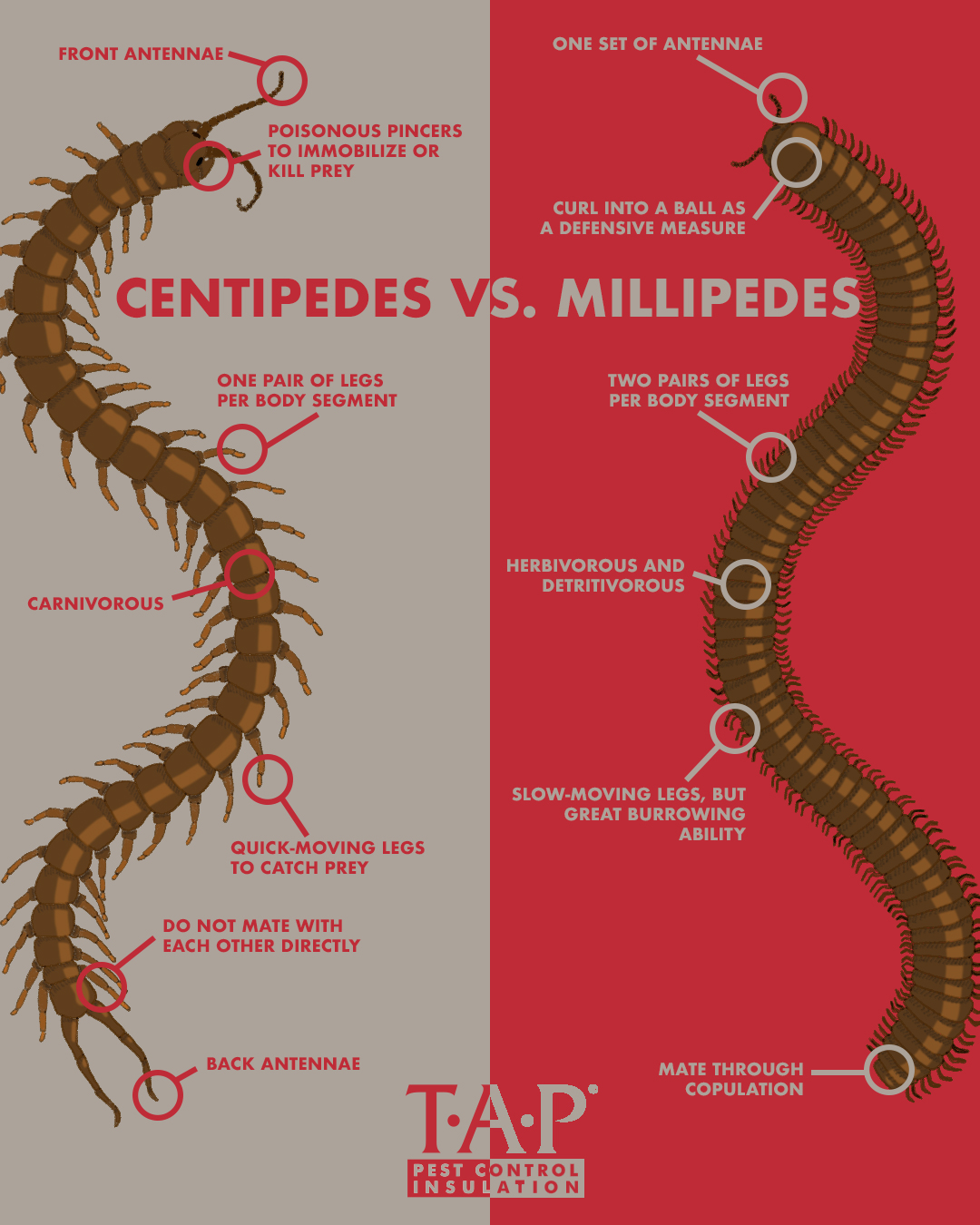This detailed infographic, titled "Centipedes vs. Millipedes," is split into two sections with distinct backgrounds: gray for centipedes on the left and red for millipedes on the right. At the top, the title is centered with an eye-catching contrast in colors – "centipedes" in red and "millipedes" in gray. The centipede on the left curves in an 'S' shape, illustrated in brown and gold, while the millipede on the right forms a backward 'S', also in brown and gold. Detailed diagrams highlight key differences between the two arthropods: centipedes have a single pair of longer legs per body segment, are carnivorous with quick-moving legs, possess front and back antennae, and utilize poisonous pincers to immobilize prey. In contrast, millipedes have two pairs of shorter legs per body segment, are herbivorous with slower-moving legs suited for burrowing, and curl into a ball as a defensive mechanism. The infographic is supplemented with bullet points and arrows detailing these features, providing an educational comparison. At the bottom, the TAP pest control insulation logo is displayed, indicating the infographic's source or sponsor.